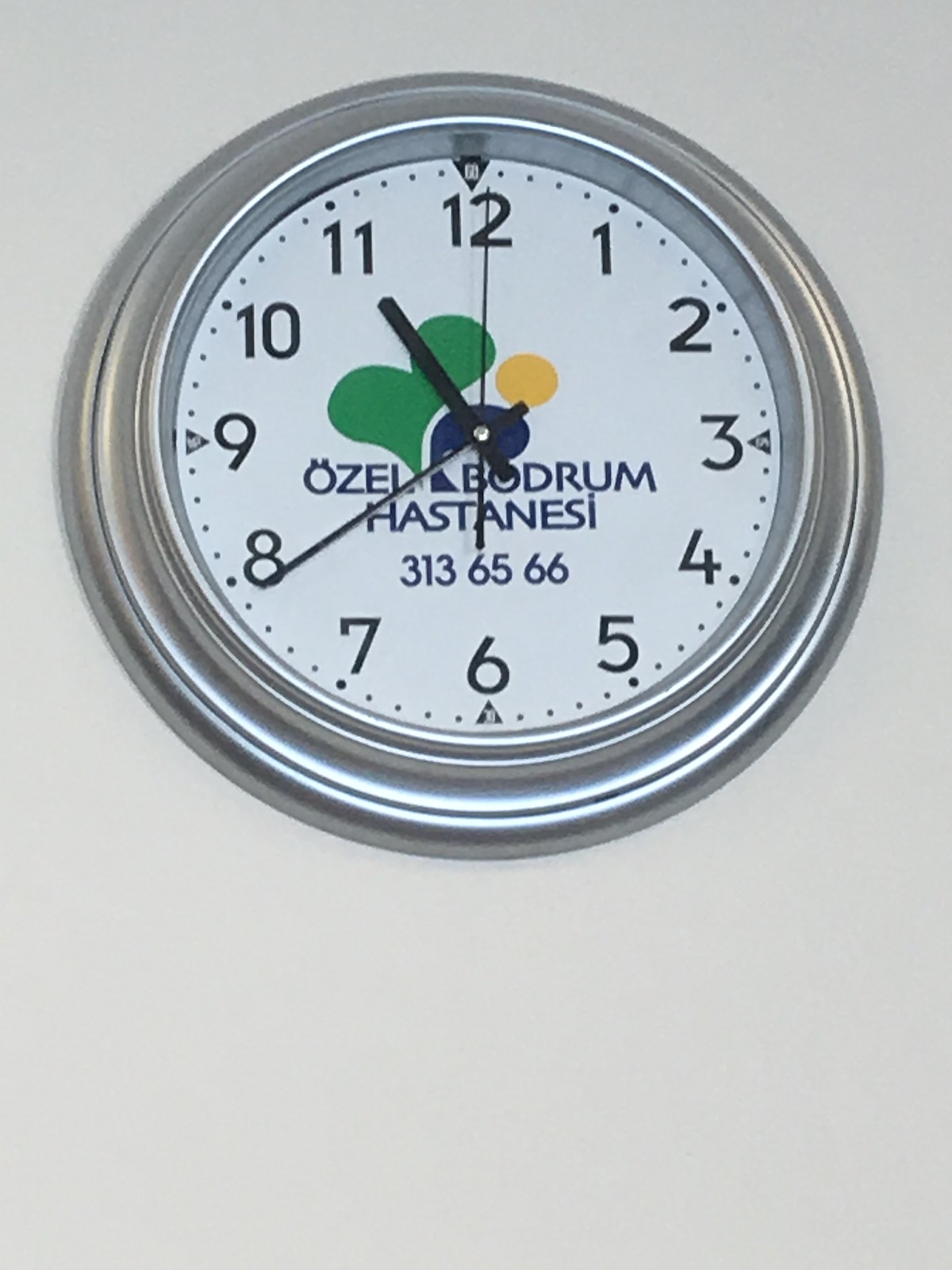The image depicts a clock mounted on a smooth, flat white wall inside a room. The circular clock has a sleek silver outer border encircling a design with various elements. Around the face of the clock, black numbers are positioned, along with several small dots and circles adorning the border. The center of the clock features text in a foreign language, specifically Turkish, spelling out "ÖZEL BODRUM HASTANESI" in blue writing. Prominently displayed above this text is a logo that includes a green heart. Additionally, the clock face showcases a blue emblem in the center and a yellow emblem towards the top right. According to the time indicated, the clock is showing approximately 11:40.